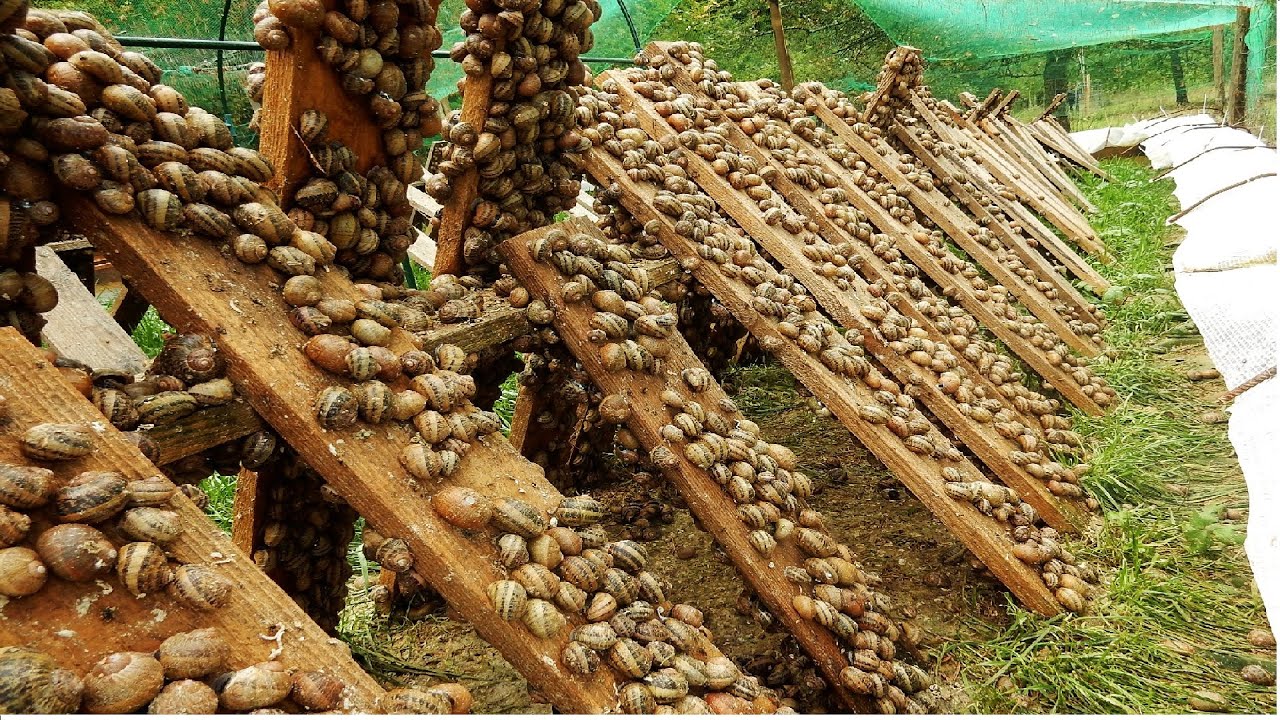This image depicts an outdoor scene in a grassy field with several wooden planks arranged at a roughly 45-degree angle, leaning against a wooden fence. These planks are covered with what seems to be an assortment of nuts or small gourds, varying in shape and size, some rounder and some more oblong. The nuts (or possibly small gourds) which appear to be coated with a sticky substance, are more densely packed near the top of the planks. To the right side of the image, a series of white bags line the fence, creating a distinct separation from the middle of the image. The scene is bright and organic, with the natural elements of wood and grass providing a rustic backdrop to the curious arrangement of these brown, oval-shaped food items.